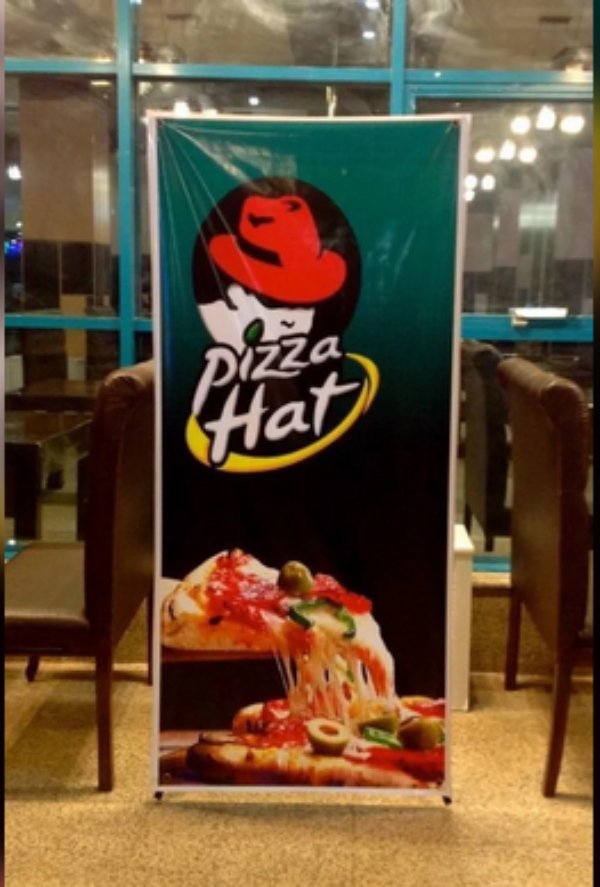The image features a zoomed-in view of a Pizza Hut advertisement prominently displayed within a restaurant setting. The advertisement takes up approximately two-thirds of the image and is centered. It showcases a teal-to-black gradient background with the Pizza Hut logo in the upper left corner. Below the logo, a person wearing a red fedora—partially covering their eyes—adds a unique twist, reinforcing the playful branding.

The focal point of the advertisement is a tempting pizza with olives, peppers, and pepperoni. A spatula is lifting a slice from the pizza, with gooey, stretchy cheese still attached, creating a mouth-watering visual. This banner is situated between two wooden tables, each flanked by brown chairs on a tan floor. In the background, large windows with teal gridded bars reflect various lights, adding depth and ambiance to the scene.